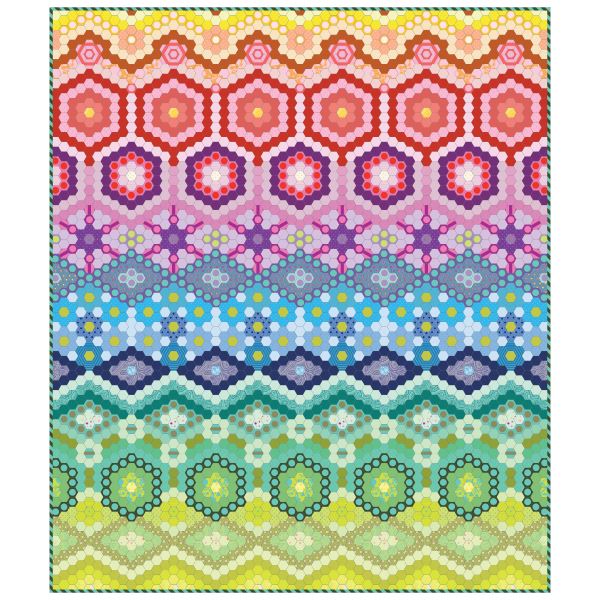The image portrays a colorful, mosaic-like quilt constructed from an array of geometric shapes including hexagons, triangles, squares, diamonds, circles, rectangles, and octagons, all meticulously organized in a harmonious, vertical striped pattern. These shapes are vividly hued, creating a visually striking spectrum that transitions from bright yellow at the top through shades of orange, red, pink, purple, blue, green, and encompasses a variety of other vibrant colors. The intricate design features rows of hexagons, with detailed color blends like red-pink-yellow and purple-red-white combinations, alongside triangles and diamond shapes in contrasting shades, showcasing a lively and ornate geometric tapestry. The quilt, standing tall in a rectangular orientation, exudes a sense of uniformity and artistic technique, with each segment exhibiting a unique yet cohesive part of the overall variegated pattern.